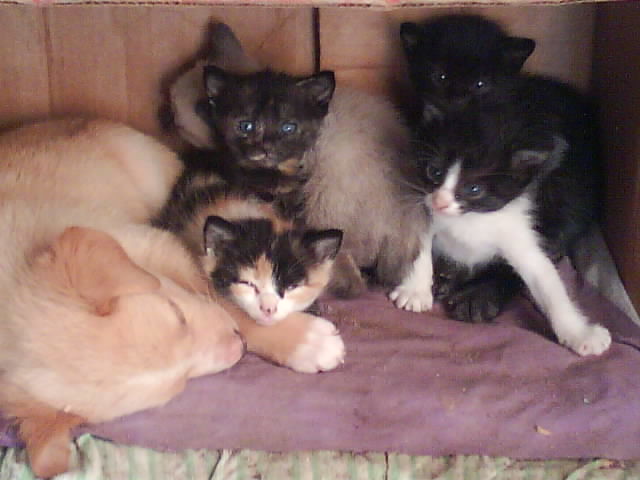This image captures a cozy, heartwarming scene set against a rustic wooden wall backdrop. Centered on a green and white plaid blanket with a purple sheet on top, lies a golden-colored puppy, possibly a young golden retriever, nestled on its right side. The puppy features a white tip on its left upper paw and slightly reddish ears. Around the puppy, five kittens are huddled together. The kitten closest to the puppy, a calico with black, white, and orange fur, adorably rests its head on the puppy’s paw. Nearby, another kitten with black and beige fur and large blue eyes peers curiously. To the right, a tuxedo kitten with a black face, a white nose stripe, and white paws is positioned in the foreground. Behind it is a solid black kitten, barely visible. In the background, a kitten with a dark face, lighter body, and striking blue eyes, resembling a Siamese, completes the cuddly assembly. The photograph, slightly blurry and taken in a non-professional setting, exudes warmth and comfort, capturing the innocent bond of these young animals.